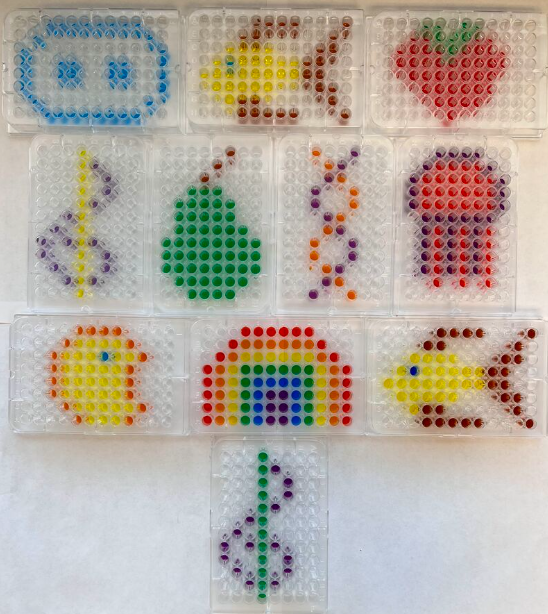The photo showcases a series of intricate arts and crafts projects laid out neatly on a white background. These projects consist of small, clear plastic grids, each containing individual compartments or bubbles. Within each compartment, colorful elements such as paint or beads have been meticulously placed to form various designs. There are three rows of grids with three pieces each, followed by four pieces in the next row, another three in the subsequent row, and a single piece centered at the bottom. The designs include a colorful fish with yellow and red fins, a green-stemmed strawberry, a jellyfish, a brightly colored rainbow featuring blue, purple, green, yellow, red, and orange, a Pac-Man figure, two musical notes—one a treble clef in purple and yellow and another in green and purple—a pear, and a pattern reminiscent of a DNA strand. While some designs feature a vibrant array of colors, others are created using just one or two shades.